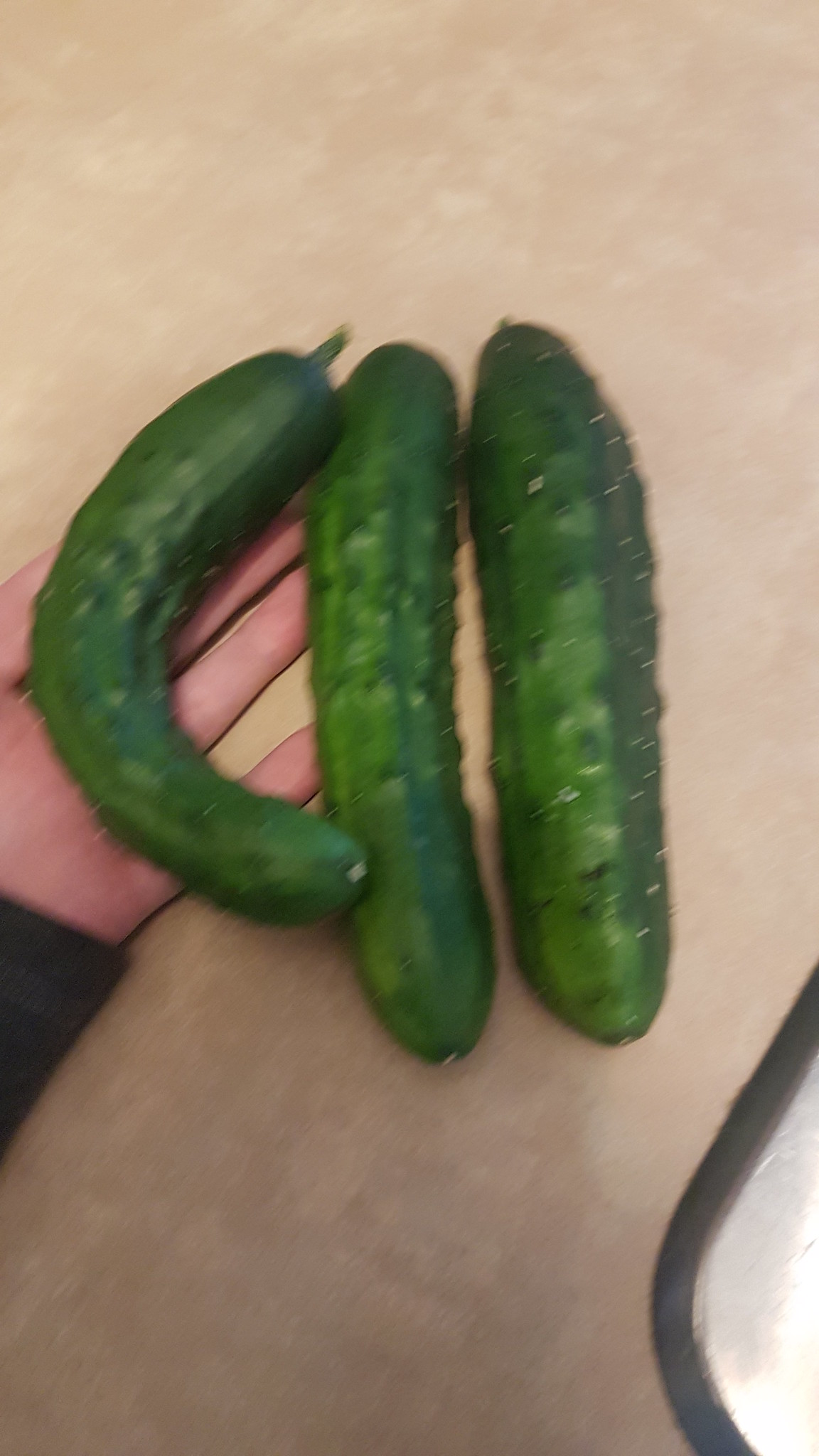In this slightly blurred image, a collection of three vibrant, dark green cucumbers is displayed against a tan, wooden platform. The cucumbers are notably bumpy, with raised dots adorning their surfaces. The leftmost cucumber is notably curved into a near C-shape, held by a person wearing a dark sweater, possibly black or dark gray. The person's hand, visibly small and fair-skinned, supports the curved cucumber, with three fingers and a thumb clearly visible while the other finger is obscured. The other two cucumbers are long and straight, lying parallel to each other. The background includes a faint black outline leading into a white area, and a tray with a black rim can be partially seen in the lower right corner. The image is taken from a top-down perspective, giving a direct view of the cucumbers.